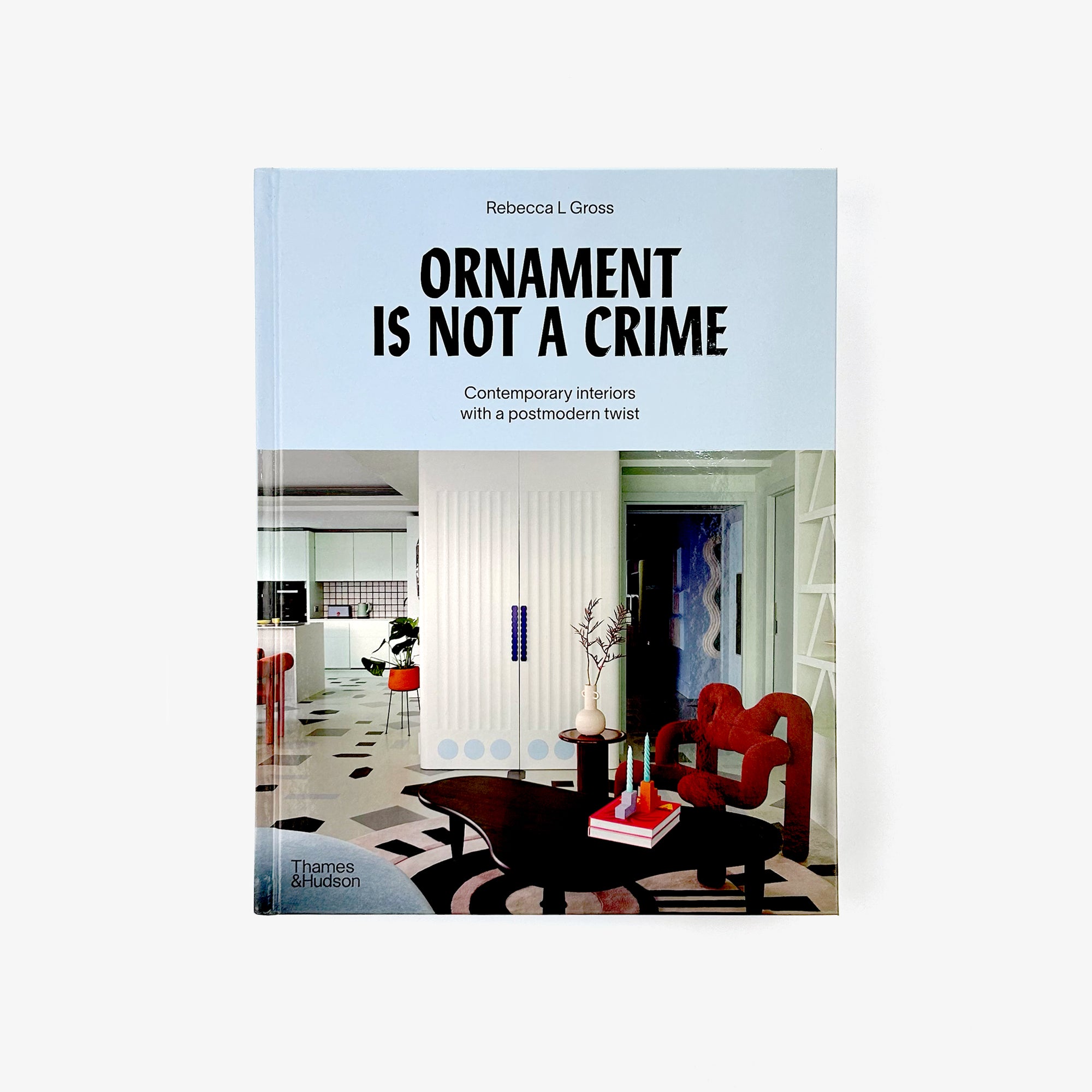The cover image of the book "Ornament is Not a Crime, Contemporary Interiors with a Postmodern Twist," authored by Rebecca L. Gross and published by Thames & Hudson, features a detailed photograph of a contemporary, postmodern interior. At the bottom of the cover, a photograph showcases a stylish house interior, specifically merging the kitchen, living room, and hallway in one cohesive space.

Dominated by a palette of blue and white, the scene includes a large white cabinet in the center, accompanied by uniquely shaped furniture. In front of the cabinet stands an abstract, modern coffee table, atop which lies a round white and black rug, two red books, and candle holders of varying colors—one red with a blue tapered candle and a light purple holder with a white candle. Adjacent to the coffee table is an oddly shaped red chair, while to its left rests a blue settee and a plant stand with a white vase filled with flowers. The right side features a white, built-in shelf for additional decor. 

The left side of the image transitions into a white kitchen, complete with countertops and cabinets that have blue circle accents at the bottom. The kitchen also features a striking checkerboard backsplash, a green coffee pot, a black coffee maker, and a silver toaster. A second plant stand with a red pot housing a cheese plant is also visible, enhancing the lively and eclectic atmosphere of the room. The overall design evokes a sense of modernistic flair with retro elements reminiscent of the 70s or early 80s, effectively capturing the essence of postmodern interior design.